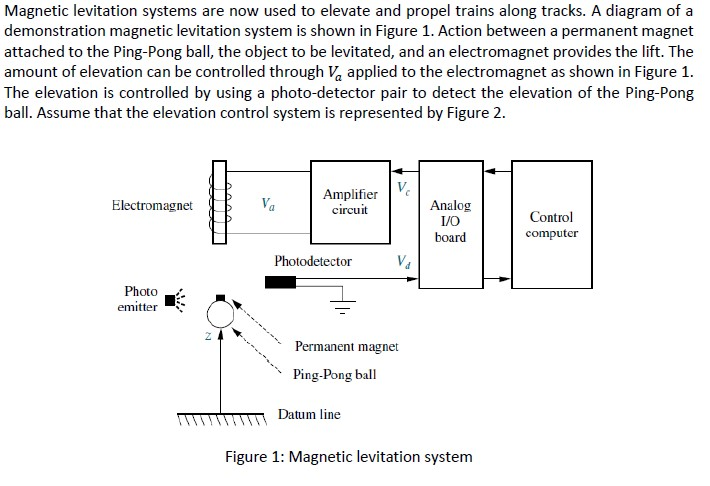The image resembles a detailed page from a science textbook, set against a white background with black text. At the top, a paragraph explains that magnetic levitation systems are currently used to elevate and propel trains along tracks. An illustrative diagram of a demonstration magnetic levitation system is shown in Figure 1. This system operates based on the interaction between a permanent magnet attached to a ping-pong ball, the object to be levitated, and an electromagnet, which provides the lift.

The amount of elevation is controlled through a variable voltage, denoted as \( V_A \), applied to the electromagnet. A photodetector pair is used to measure the elevation of the ping-pong ball, to adjust \( V_A \) accordingly. Assume the elevation control system references Figure 2, which is not provided.

In the diagram (Figure 1), the top-left corner features an electromagnet, connected through various components: first an amplifier circuit, followed by an analog input-output (I/O) board, and finally a control computer. These elements are linked sequentially by lines. Below this setup, a photodetector is connected, and beneath it is a photo emitter located on the left side. The diagram also includes labels such as \( V_C \) and \( V_D \) with arrows indicating their directions.

Towards the bottom, the ping-pong ball with a permanent magnet on top is depicted, levitating above a horizontal line called the datum line. The ball is centrally positioned with dashed arrows pointing up from the sides, one labeled permanent magnet and the other ping-pong ball. At the very bottom, the diagram is labeled as Figure 1 - Magnetic Levitation System.